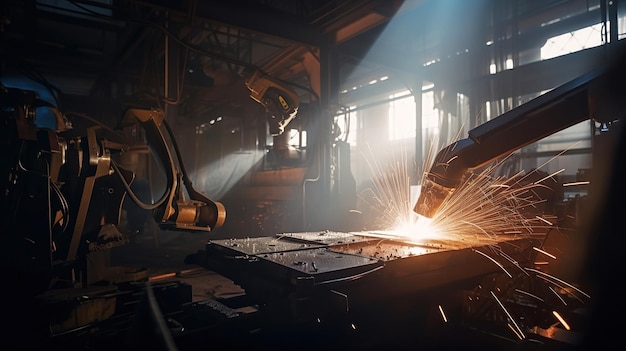In a dimly lit factory space, illuminated subtly by a skylight and large windows at the back, two robotic arms are engaged in a welding operation. The scene features dark metal pieces scattered around a table in the foreground. The robotic arm on the right is actively welding, sending a shower of sparks into the air as it works on a steel plate. Its counterpart on the left stands idle, positioned away from the ongoing project. The setting, reminiscent of a workshop or garage, is bathed in minimal light, emphasizing the bright sparks from the active welding process amidst the otherwise shadowy environment. The dark ambiance of the room contrasts sharply with the vivid burst of welding activity, highlighting the precision and functionality of the robotic arms reminiscent of human limbs in their movements.